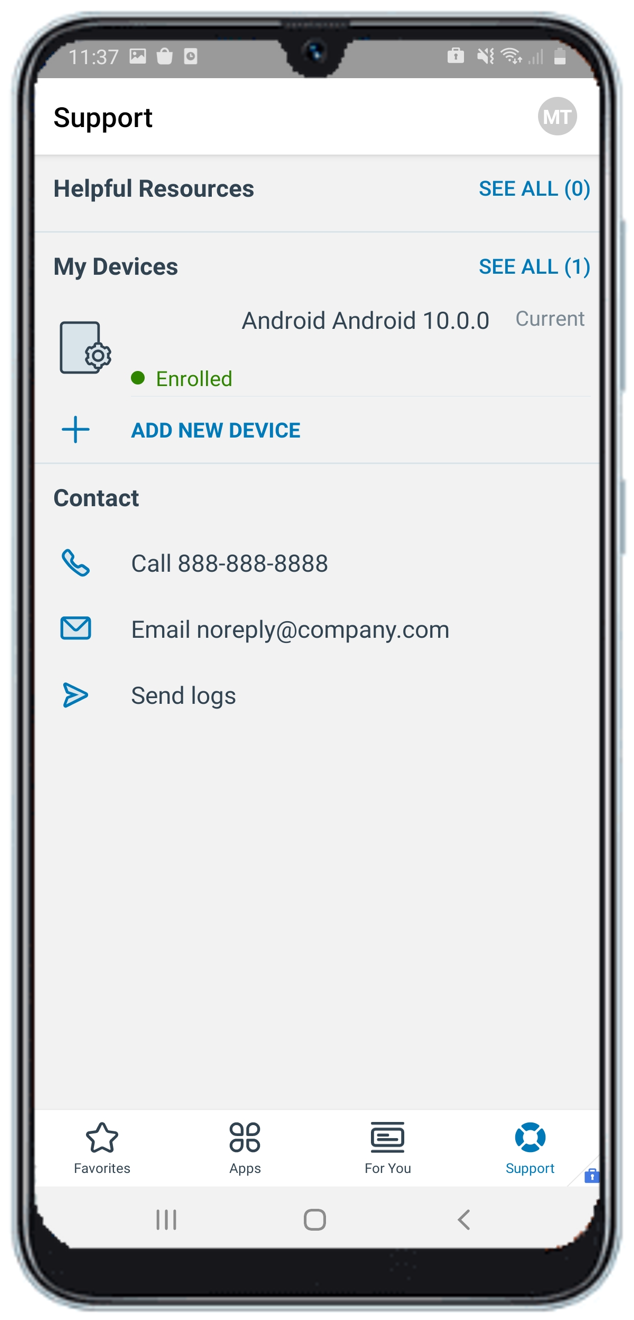This image showcases a detailed interface of a smartphone screen. At the top, the screen displays the time "11:37" in gray font. Accompanying the time, there is a series of icons including a shopping bag, an indiscernible rectangular image, a lock, an unclear element, a Wi-Fi symbol, ascending bars representing signal strength, and a battery icon.

Beneath the time, there is a prominent white rectangle with the word "Support" written on it. Below this, a gray circle marked "MT" is visible, followed by a gray rectangle with further information.

The left section beneath the "Support" banner offers "Helpful Resources" with a button labeled "See All (0)" in blue on the right. Below it, under the "My Devices" section, there’s an option to "See All (1)" also in blue. A description below this reads "Android 10.0.0 current," accompanied by an image of a document with a gear icon and a green dot stating "Enrolled."

A blue plus sign with "Add new device" written next to it is prominently displayed. Following this, there are options labeled "Contact" featuring a phone icon next to the number "888-888-8888," an envelope icon with "no-reply@company.com," and a paper airplane icon indicated by "Send logs."

Further down the interface, a blank space precedes another white rectangle housing a star icon labeled "Favorites" and a flower-like icon named "Apps." There’s a gray outlined rectangle with two lines inside and text beneath reading "For You." Further, there is a blue circle with four breaks enclosing a white dot in the center, labeled "Support." To the right of this circle, three vertically aligned lines, a square, and a left-pointing arrow complete the visual elements of this phone interface.